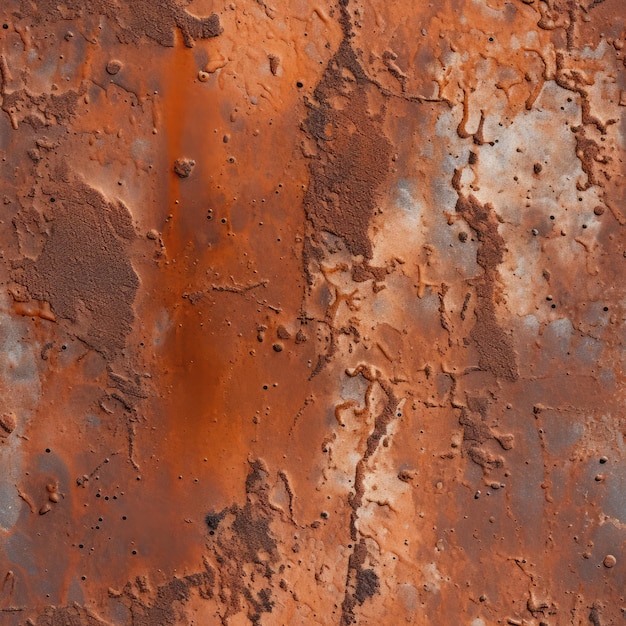The image displays a surface that combines elements of both rusting metal and stone under natural outdoor light. The predominant color is a coppery, rust-brown with shades of orange, reminiscent of decaying iron. The textured surface features numerous small black holes and bubbles indicative of rust and weathering. There are various elevations and indentations, creating an uneven, gravelly texture. The color palette includes not only rust and orange but also light blues, grays, and some dark, burnt patches. This intricate mix of shades and textures, with its pockmarked, cracking, and cresting surface, could almost be mistaken for a piece of abstract art.